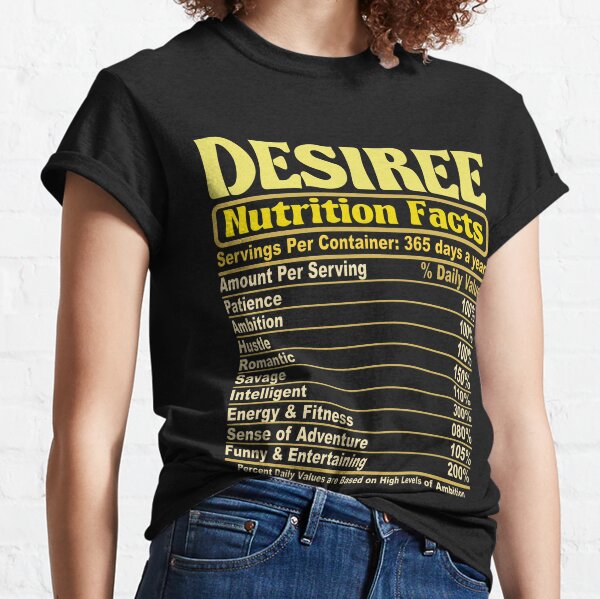The image depicts a photograph of a female model wearing a black, short-sleeved crew neck t-shirt with blue jeans, set against a plain white background. The model is visible from the waist to the lower neck, with red hair captured in the frame. The t-shirt features detailed text in yellow and white that reads "Desiree" at the top, followed by "Nutrition Facts." The text humorously lists various attributes with their respective values, including: "Servings per container: 365 days a year," "Amount per serving: Patience 100%, Ambition 100%, Hustle 100%, Romantic 150%, Savage 110%, Intelligent 300%, Energy and Fitness 80%, Sense of Adventure 105%, Funny 200%, Entertaining 200%." The daily values are humorously exaggerated to emphasize high levels of these qualities.